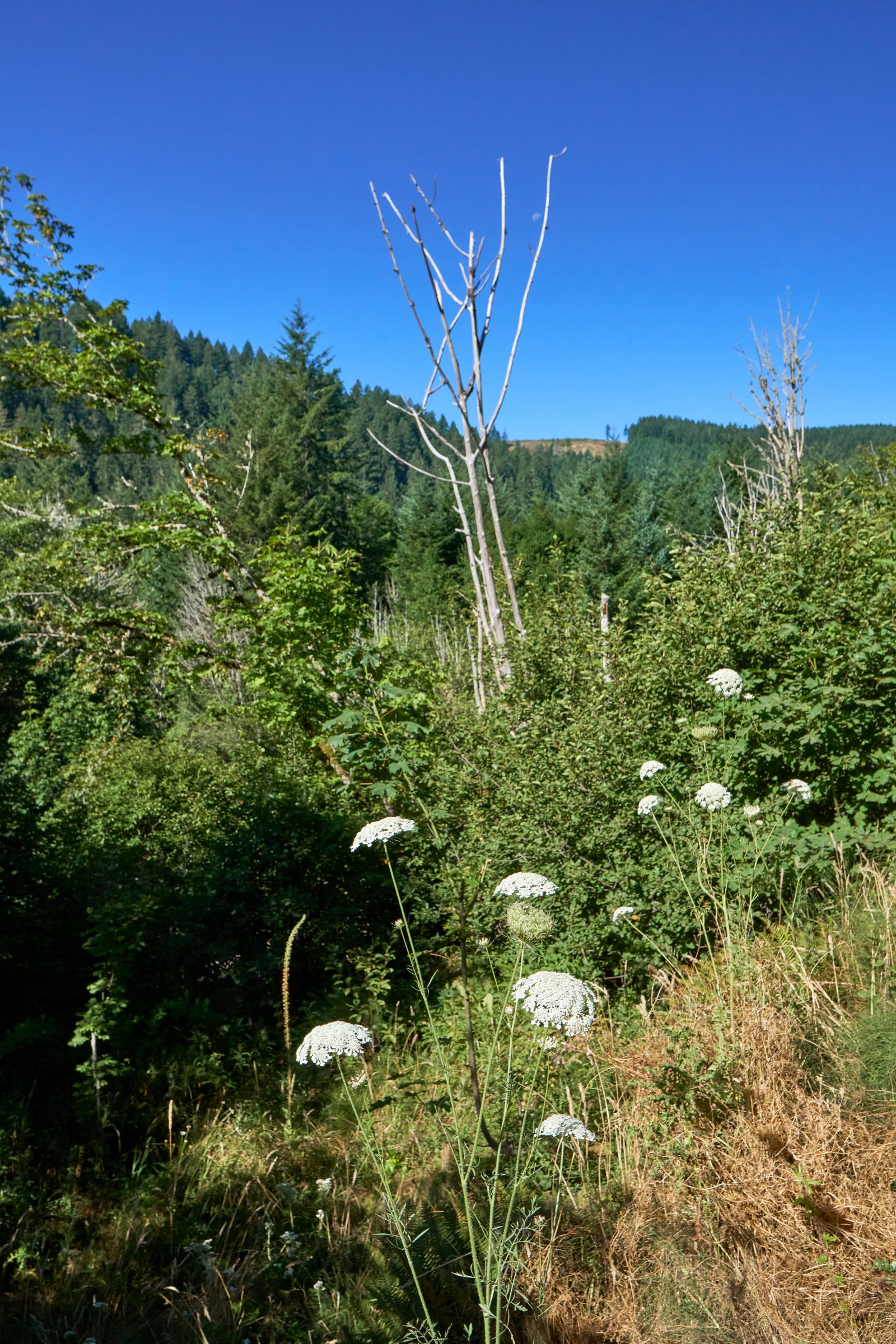The image is a vertically aligned outdoor photograph capturing a wild, untamed landscape. The foreground is dominated by tall green and brown grass, interspersed with clusters of Queen Anne's lace, identifiable by their long thin green stems and delicate white flower heads that resemble the shape of mushrooms. There are about four or five of these flowers centrally located at the bottom, with a similar number off to the right side. Interspersed among the flowers are some tall bushes and brown patches of dried grass.

In the center of the image, a leafless, dead tree stands prominently with its gray branches stretching upwards. Higher up in the picture, the background transitions to a dense hill covered with dark green conifers. These tall pine trees form a stark contrast against the clear blue sky that dominates the top portion of the image. No clouds are visible, suggesting a bright, clear daytime setting. The overall composition is vivid and detailed, highlighting the natural, unspoiled beauty of the area.